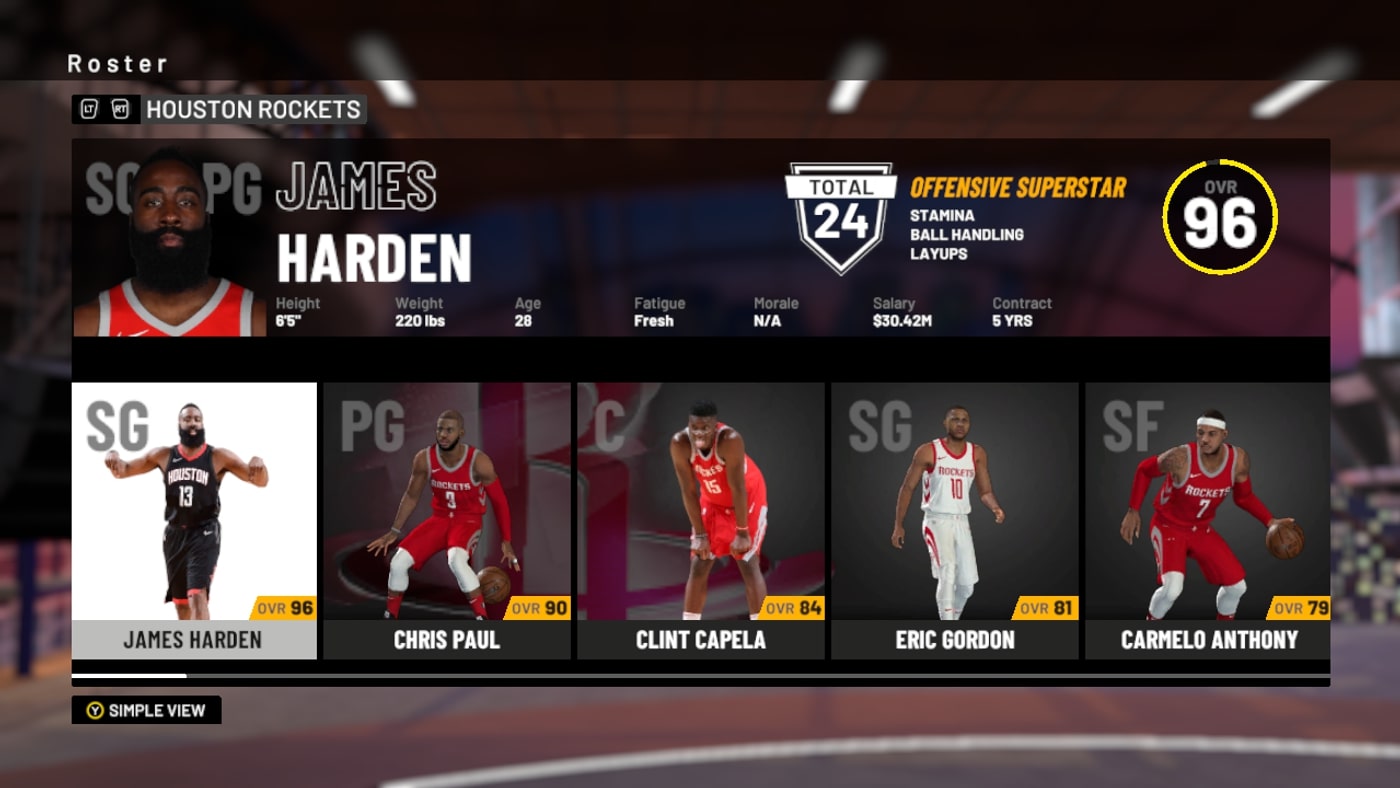This screenshot from a sports video game captures the user interface set against a blurred background of a dimly lit basketball arena. The arena features three distinct strips of light at the top, providing minimal illumination amidst the dark setting. The game interface itself is detailed and multi-layered.

At the top, a mostly translucent black header spans the width of the screen, with a single line of white text in the bottom left that reads "Roster." Beneath this header is a two-toned box, dark gray on the right and black on the left. Overlaying the black portion are two nearly rectangular white symbols angled inward. The left symbol is labeled "LT" while the right is labeled "RT."

The main overlay, a dark translucent rectangle, contains detailed information. This section is divided into several parts:

1. **Player Image and Basic Information**:
   - A clear picture of James Harden, identifiable by his prominent black beard and sleeveless red Houston Rockets jersey, occupies the top-left corner.
   - To the right, detailed information is listed:
     - Name: James Harden
     - Title: Biddy That (category information in gray and the specific detail in white)
     - Height: 6 feet 5 inches
     - Weight: 220 pounds
     - Age: 28
     - Fatigue: Fresh
     - Morale: Not Applicable
     - Salary: $30.42 million
     - Contract: 5 years

2. **Player Ratings and Attributes**:
   - In the top-right corner, a black circle with a yellow outline displays "OVR 96" in white text, denoting an overall rating of 96.
   - Below this, in orange text, reads "Offensive Superstar."
   - Following this, a list of skills is shown in white text: "Stamina, Ball Handling, Layups."

3. **Additional Icons and Player Information**:
   - To the left of the skill list, a shield-shaped icon with a black center and white outline contains the number "24." A white bar across the icon reads "TOTAL" in black text.

Beneath this primary section, smaller images representing five other players are displayed, indicating a broader roster or team lineup.

This detailed interface provides comprehensive information about James Harden along with supplementary visuals and data points, all integrated into the game's visually dark yet dynamic backdrop.